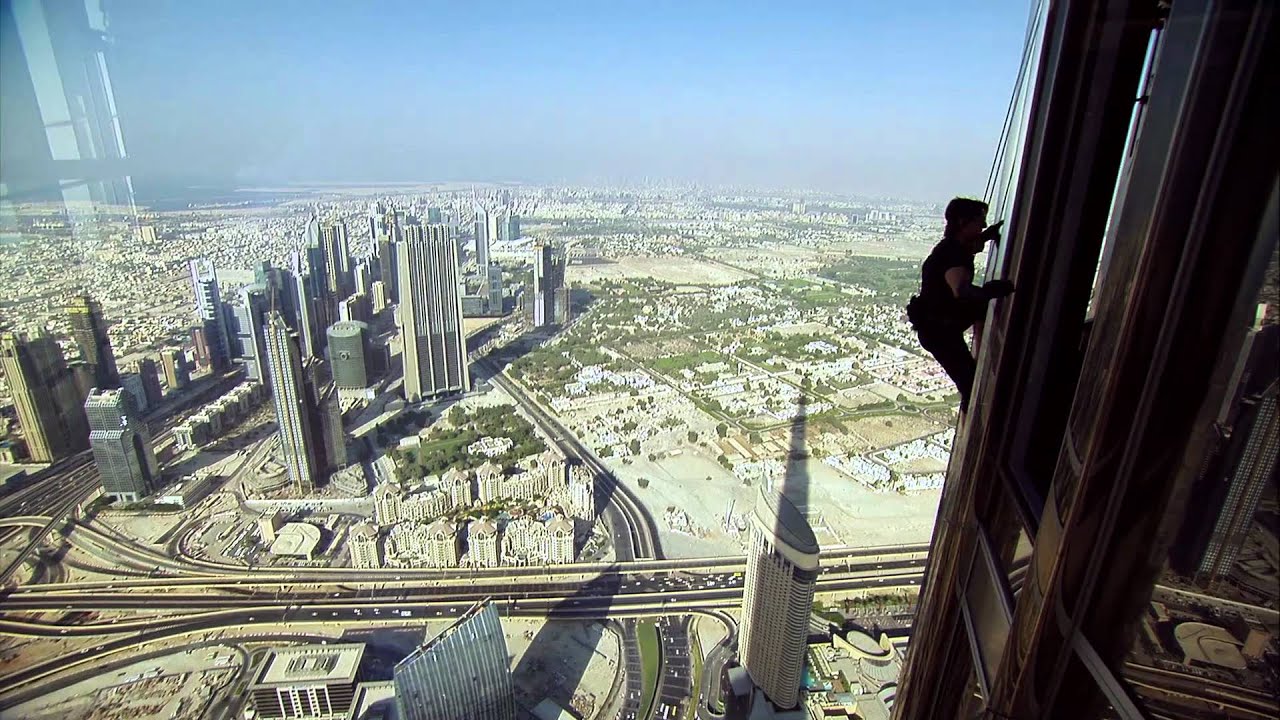This stunning aerial photo captures the dizzying height and grandeur of a modern desert city, likely in the United Arab Emirates, possibly Dubai. Taken from inside one of the city’s tallest skyscrapers, it reveals a man scaling the exterior wall, suspended by ropes and tethers. The climber, who might be a window washer or perhaps engaged in a thrilling stunt, is dressed in all black and cast in shadow, his form silhouetted against the sprawling urban landscape.

In the left-hand corner of the image, the reflective glass of the building adds an extra layer of depth, while the right side shows the building's shadow. The city's skyline beneath features a dense cluster of tall skyscrapers and variously shaped buildings, including rectangular and a few cylindrical structures. Far below, the network of highways weaves through sparse patches of greenery and desert-like terrain, stretching toward a distant, slightly hazy horizon under a light blue sky. The cityscape combines both modern urban planning and natural elements, offering a stark contrast between the towering, sleek buildings and the more barren desert ground.